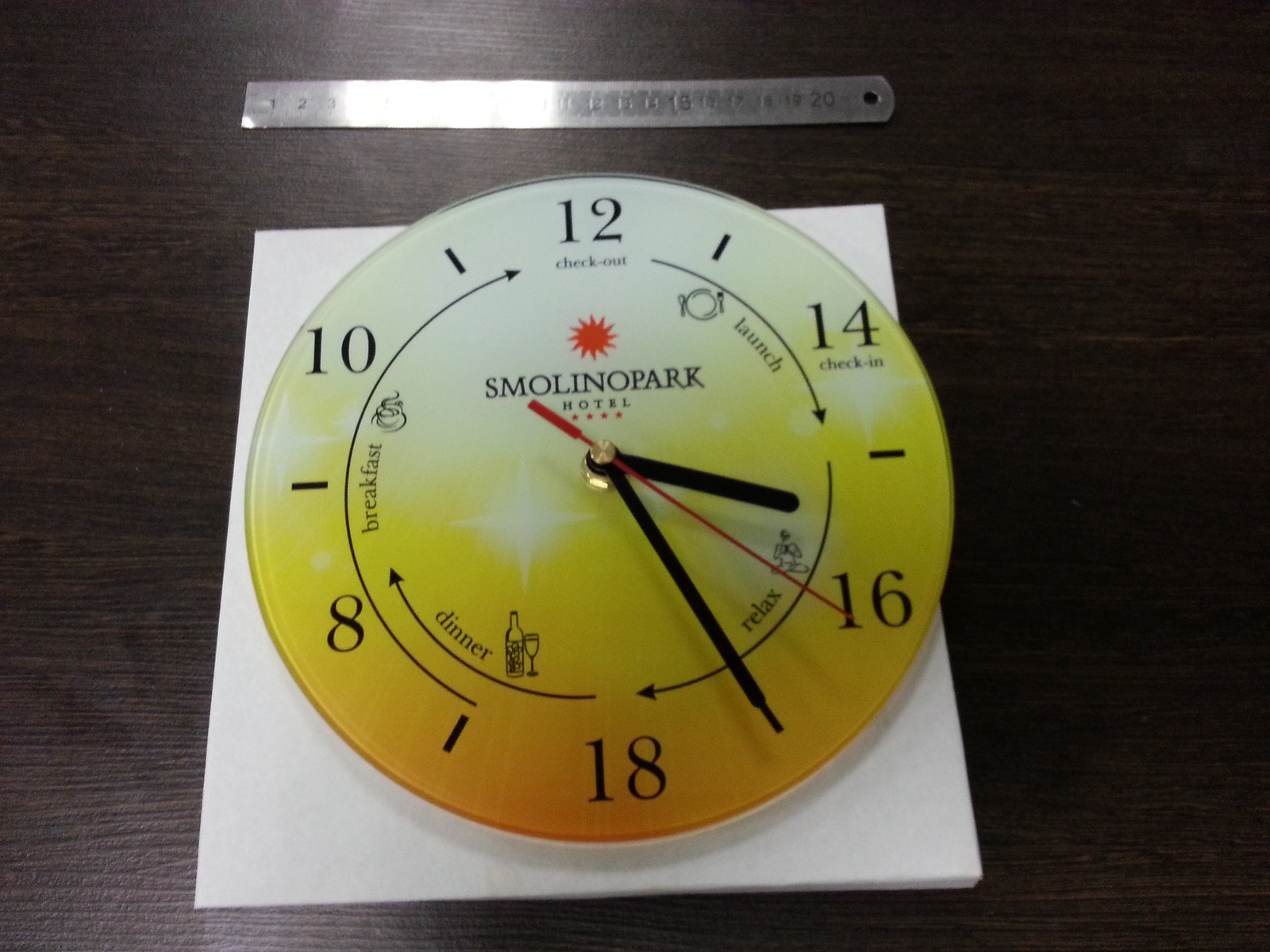A vivid image of a decorative desk clock situated at the Smolino Park Hotel. The clock, prominently placed on a desk with a rich chocolate brown finish, rests atop a protective white foam padding. Its design is vibrant, starting with an orange base that gradients through yellow to white at the top. Scattered around the clock face are small, white stars that add a whimsical touch. The clock face features both numerical and word markers: 12, 14, 16, 8, and 10 are complemented by labeled segments, guiding guests through their day with indications for "check out," "lunch," "relax," "dinner," and "breakfast." Currently, the solid black hour and minute hands, along with a striking red second hand, point to 15:25 (3:25 PM), signifying the "relax" timeframe.